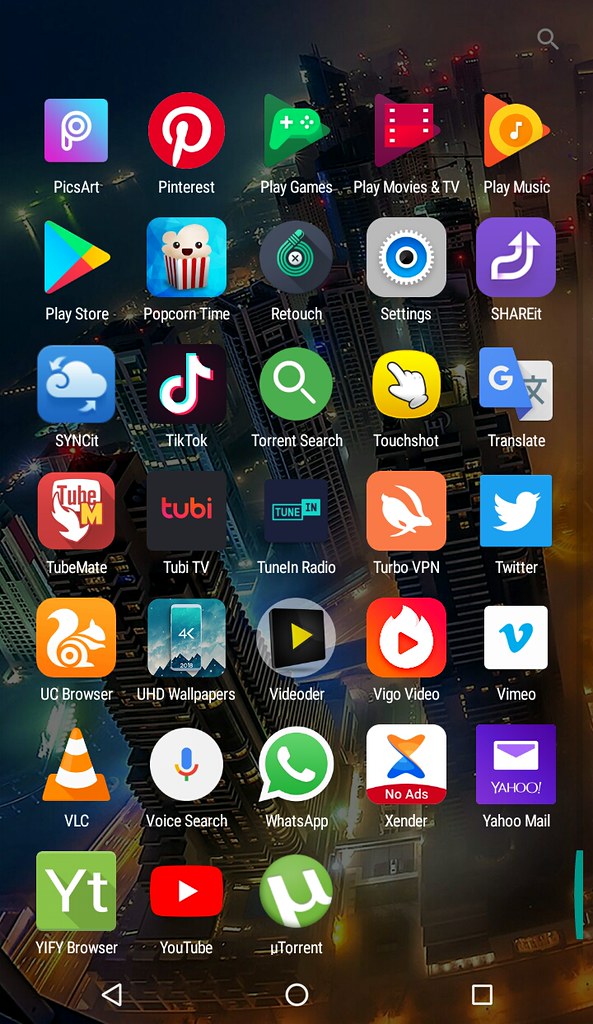This image depicts a screenshot of an Android home screen set against the backdrop of a dark, aerial view of a city taken at night, giving off a moody, Batman-esque vibe. The black skyscrapers loom in the background, contributing to the overall dark theme. The screen is populated with a variety of apps, all arranged alphabetically from left to right, five icons per row, and scattered without any folders.

The visible apps include, in order: PicsArt, Pinterest, Play Games, Play Movies & TV, Play Music, Play Store, Popcorn Time, Retouch, Settings, Share, Sync, TikTok, Torrent Search, Touch Shot, Translate, TubeMate, Tubi TV, TuneIn Radio, Turbo VPN, Twitter, UC Browser, Wallpapers, Video, Vigo Video, Vimeo, VLC, Voice Search, WhatsApp, Xender, Yahoo Mail, YIFY Browser, YouTube, and uTorrent.

At the top right corner of the screen is a small search bar. At the bottom, the standard Android navigation buttons are visible: a back button, a circle button, and a square button.